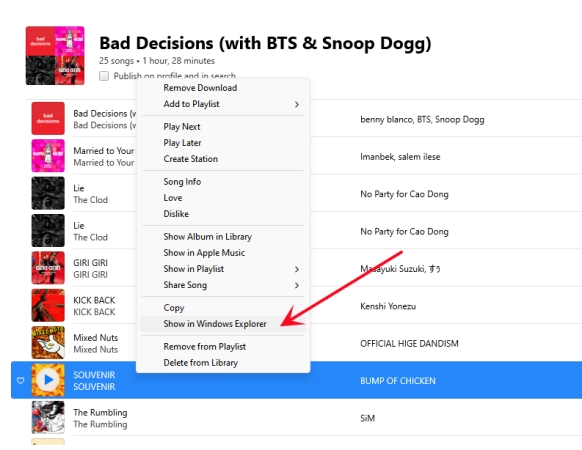The image depicts a section of an entertainment website. In the top left corner, there's an icon resembling a record album divided into four squares. Next to the icon, the text "Bad Decisions" is prominently displayed in bold black font. Adjacent to this, in parentheses, it reads "With BTS and Snoop Dogg." Directly below, in smaller text, it specifies "25 songs, 1 hour, 28 minutes." 

Beneath this description is a checkbox labeled "publish," but the remainder of the sentence is obscured by an overlay box containing various options. The options listed in the overlay include "remove download," "add to playlist," with a directional arrow pointing right, and "play next," among others. Additional choices listed include "play later," "create station," "song info," "love," "dislike," "show album in library," "show in Apple Music," "show in playlist," "share song," "copy," "show in Windows Explorer," marked with a long red arrow, "remove from playlist," and "delete from library."

Below this overlay, there are various album titles, including "Lie," "The Clod," repeated several times, and "Gary Gary" also repeated. Notable titles like "Kick Back," "Mixed Nuts," and "Souvenir" appear, with "Souvenir" highlighted in blue alongside the band name "Bunk Chicken." Finally, the titles "The Rumbling" appear twice consecutively.